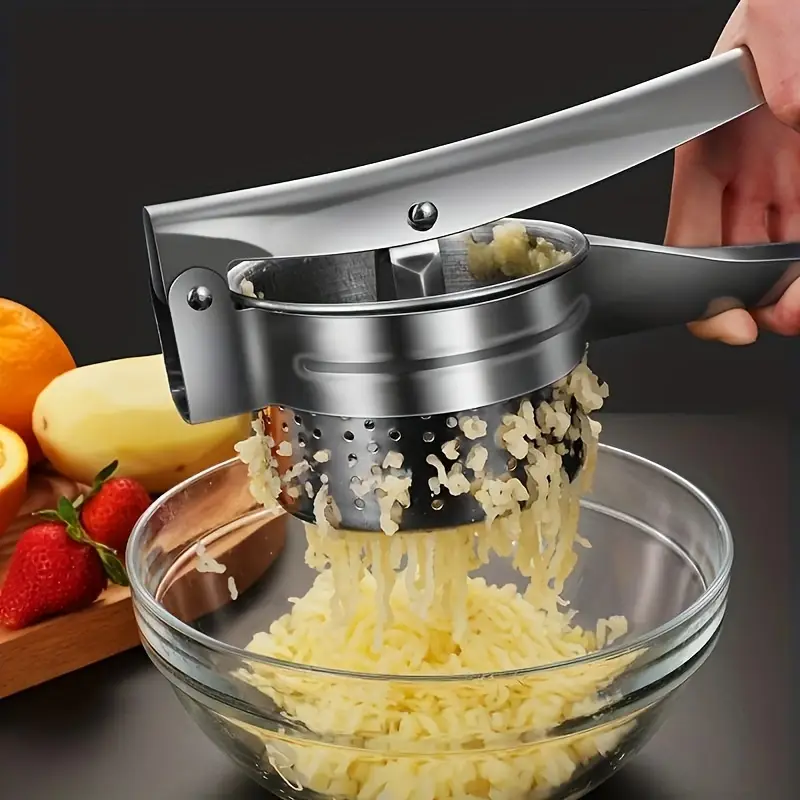The image depicts a professionally shot scene with a dark background and a gray tabletop, illuminated with high-quality lighting. It focuses on a hand in the upper right corner holding a steel ricer, squeezing riced potato into a clear glass bowl that is about one-third full. To the left, a wooden serving board displays a peeled potato, a halved orange, and several strawberries. The attention to detail, particularly on the ricer and the bowl, highlights the meticulous setup typical of professional food photography.